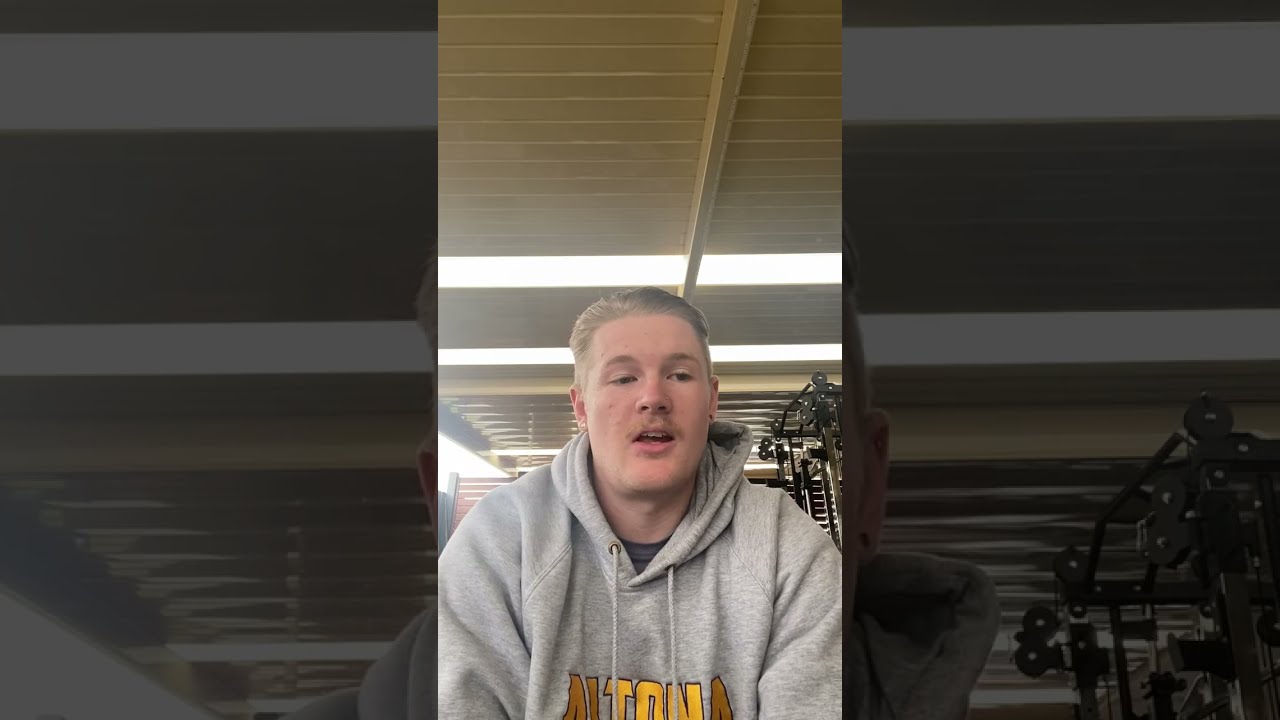The photograph divides into three vertical sections, with the first and third sections showing darkened close-ups of the central section. In the middle section, a young man with dirty blonde or light brown hair and a small mustache is the focal point. He is captured mid-sentence, his mouth slightly open as if talking. The man is wearing a heather gray hoodie adorned with yellow or golden lettering, which is difficult to fully decipher but partially reads "Tona." Strings dangle from the hood, indicating it's a hoodie. He has a piercing on his left ear. The background suggests an indoor gym setting with various machines and equipment visible behind him, illuminated by white fluorescent lights attached to a cream-colored ceiling. The room is well-lit and spacious, emphasizing the gym environment further.